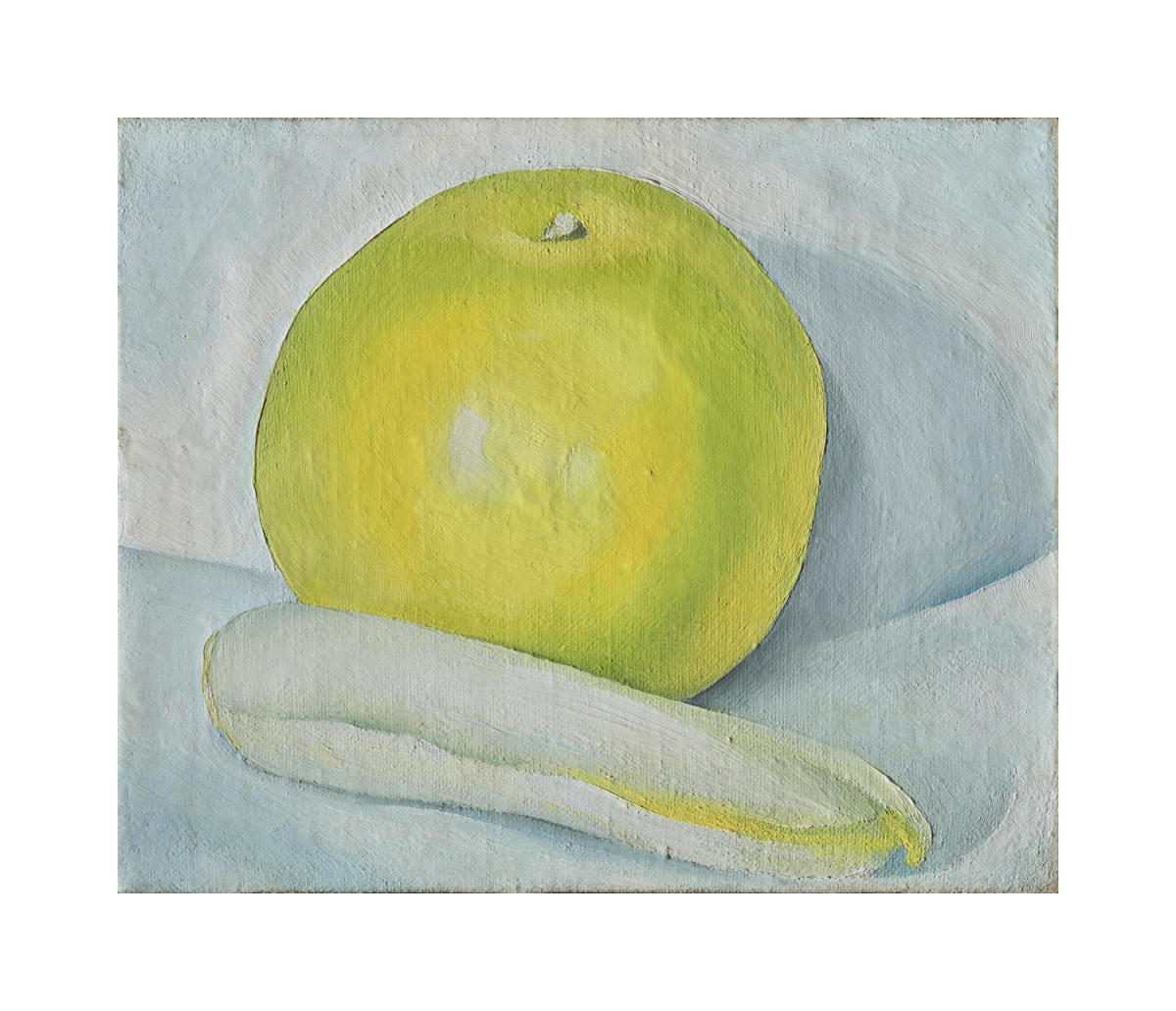This is a photograph of a painting depicting a green, partially disfigured fruit with a small white stem emerging from its top. In front of this fruit, there is a cucumber-shaped object rendered in a pale, off-white hue with subtle yellow undertones. The backdrop is a blend of bluish-white tones with gray shadowing, adding depth and texture. Despite being slightly blurred, the image reveals an artistic application of shadowing, highlighting the contours and imperfections of the subjects.